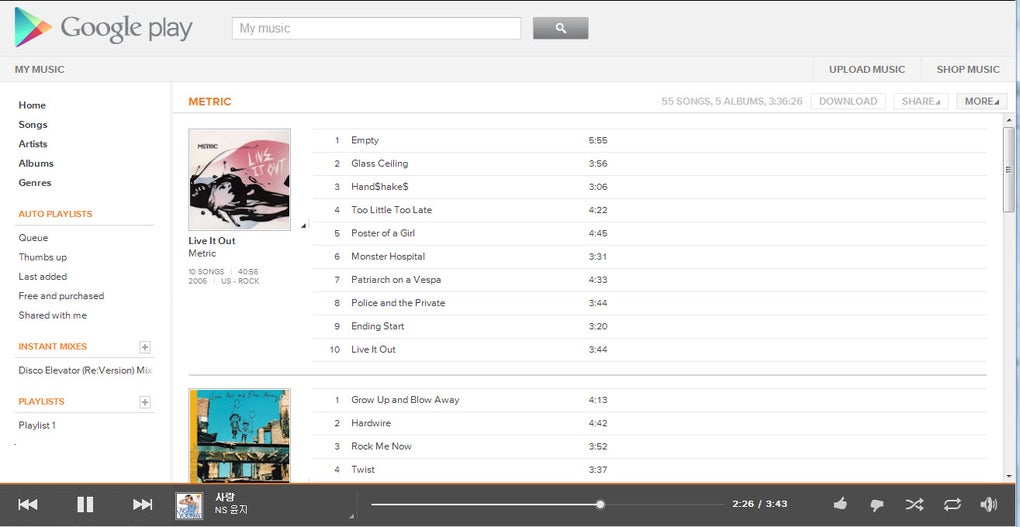The image portrays a webpage from the Google Play Music service. In the upper left-hand corner, the Google Play logo is prominently displayed. On the left side, there is a navigation menu vertically aligned with options such as Home, My Music, Songs, Artists, Albums, Genres, Auto Playlists, Queue, Thumbs Up, Last Added, Free and Purchased, Shared with Me, and Instant Mixes. 

At the bottom of the page, there is a black bar indicating that a song is loaded, with a visible pause button suggesting that music playback can be controlled from this section.

The main body of the webpage features music content, starting with an album by the band Metric, accompanied by its cover art. The album cover is pink, and underneath, there is a list of songs along with their durations. Further down, another album is featured, with a greenish cover, also listing numerous songs in a similar format.

At the top right corner of the page, there are options to upload music and shop for music, along with a 'More' button for additional features or settings.